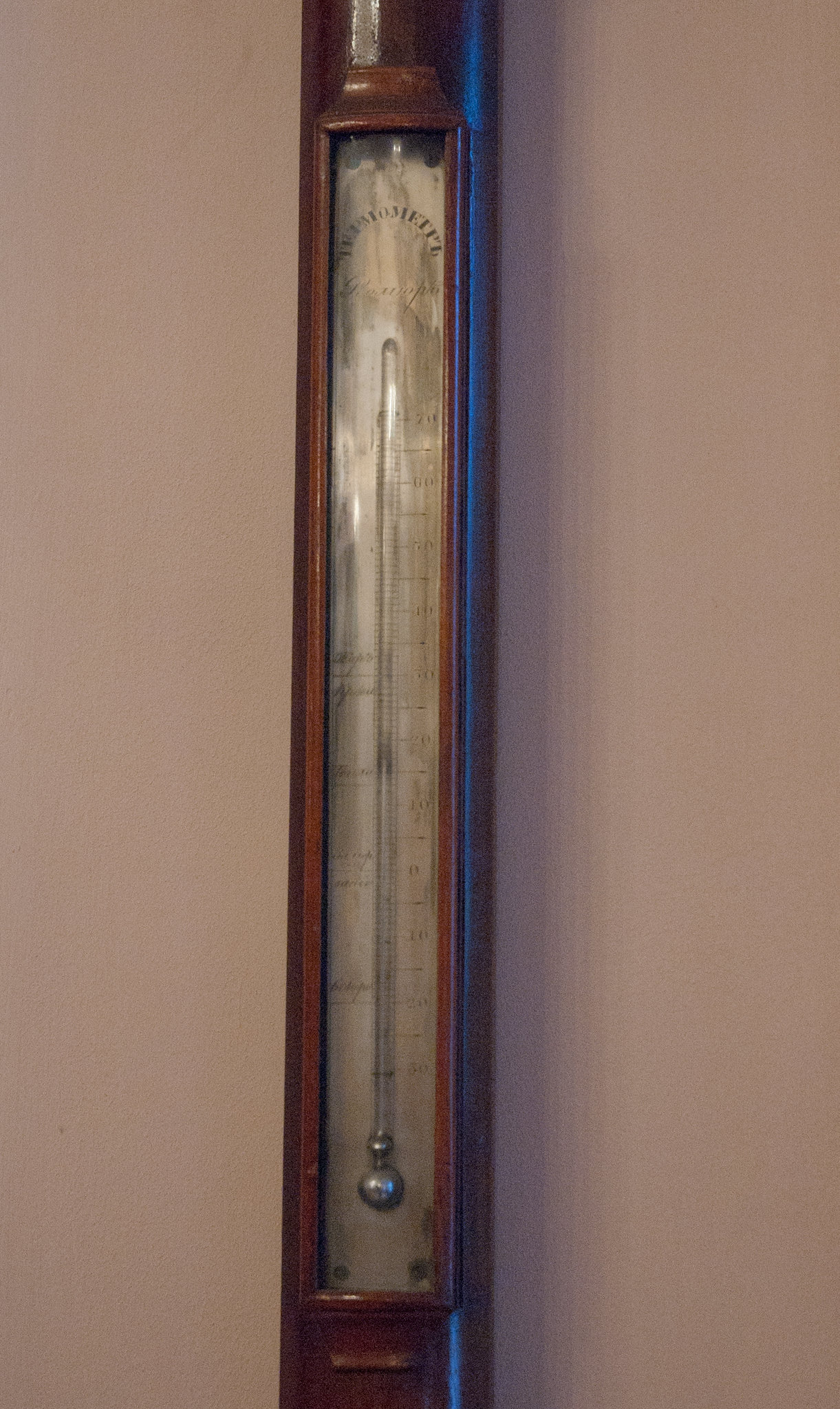The image features a vintage wall-mounted thermometer encased within a slender, wooden frame. The thermometer, which is notably longer and narrower than typical wall thermometers, contains a glass tube filled with a silver-colored liquid, likely mercury. Faint, but distinguishable, text at the top of the device seems to spell out "thermometer." The thermometer displays temperature readings with scale markings on both sides of the tube; one side presumably indicates Fahrenheit, while the other denotes Celsius. A protective glass cover shields the thermometer, reflecting a subtle blue glare of light along its left side. The wooden frame and glass create a visible vertical shadow on the white to gray wall behind it, emphasizing the thermometer’s elongated shape.